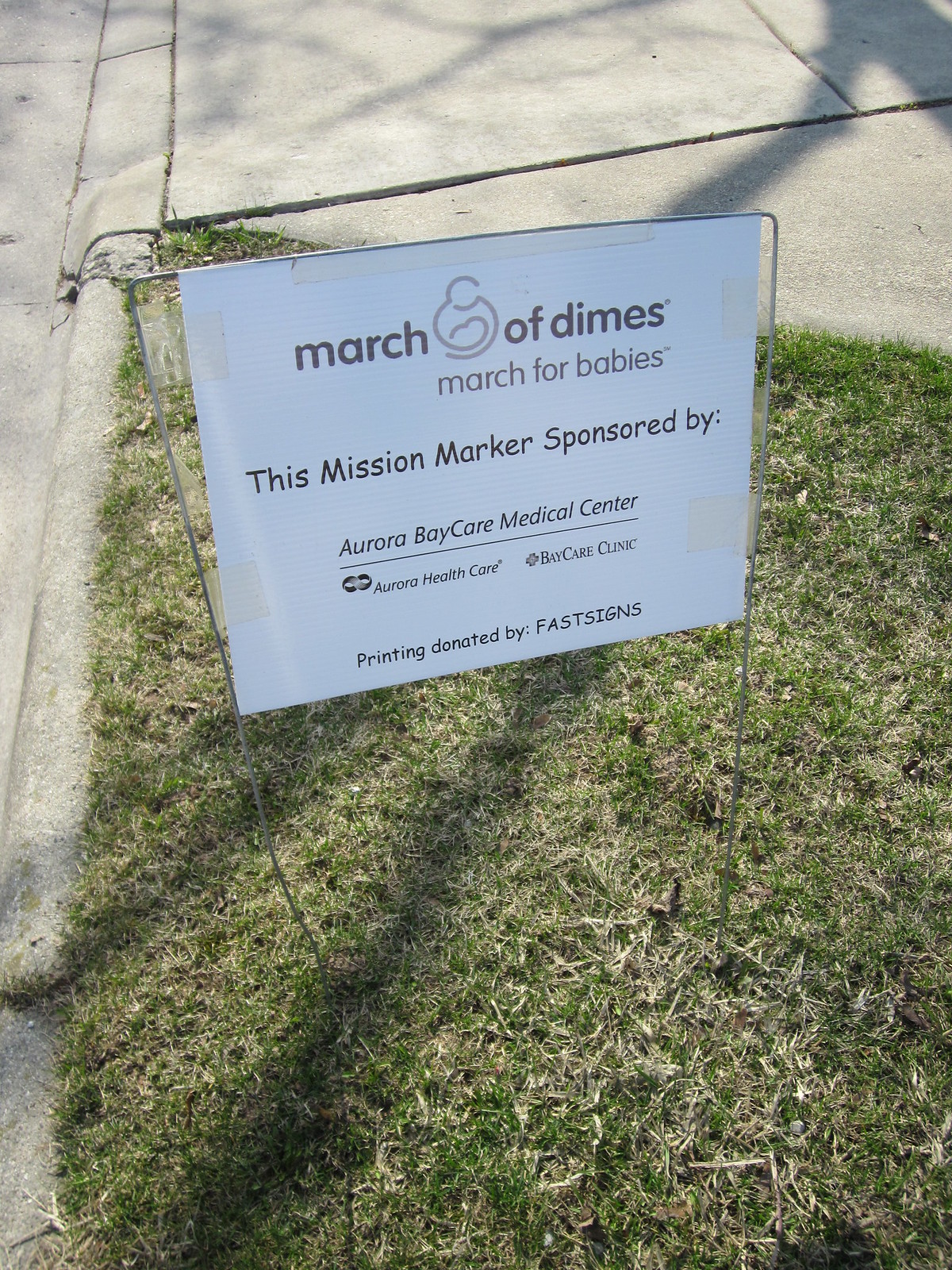The image depicts a white sign on a grassy lawn, mounted using thin metal rods that anchor it into the ground. The grass around the sign is a mix of green and patches of dead, yellowing areas. The sign reads in dark brown or maroon lettering "March of Dimes, March for Babies," with the March of Dimes symbol positioned between the words "March" and "of." Beneath this, the sign states, "This Mission Marker Sponsored By," followed by "Aurora BayCare Medical Center," a line, then "Aurora Health Care, BayCare Clinic," and "Printing Donated By Fast Signs" in descending order. The text is a combination of sans serif and Comic Sans fonts. The sign is visibly held together with transparent tape. Surrounding the grassy area is a sidewalk made of cement, visible at the top and left parts of the image, where shadows of tree branches stretch across the pavement, indicating it is daytime with a clear sky.